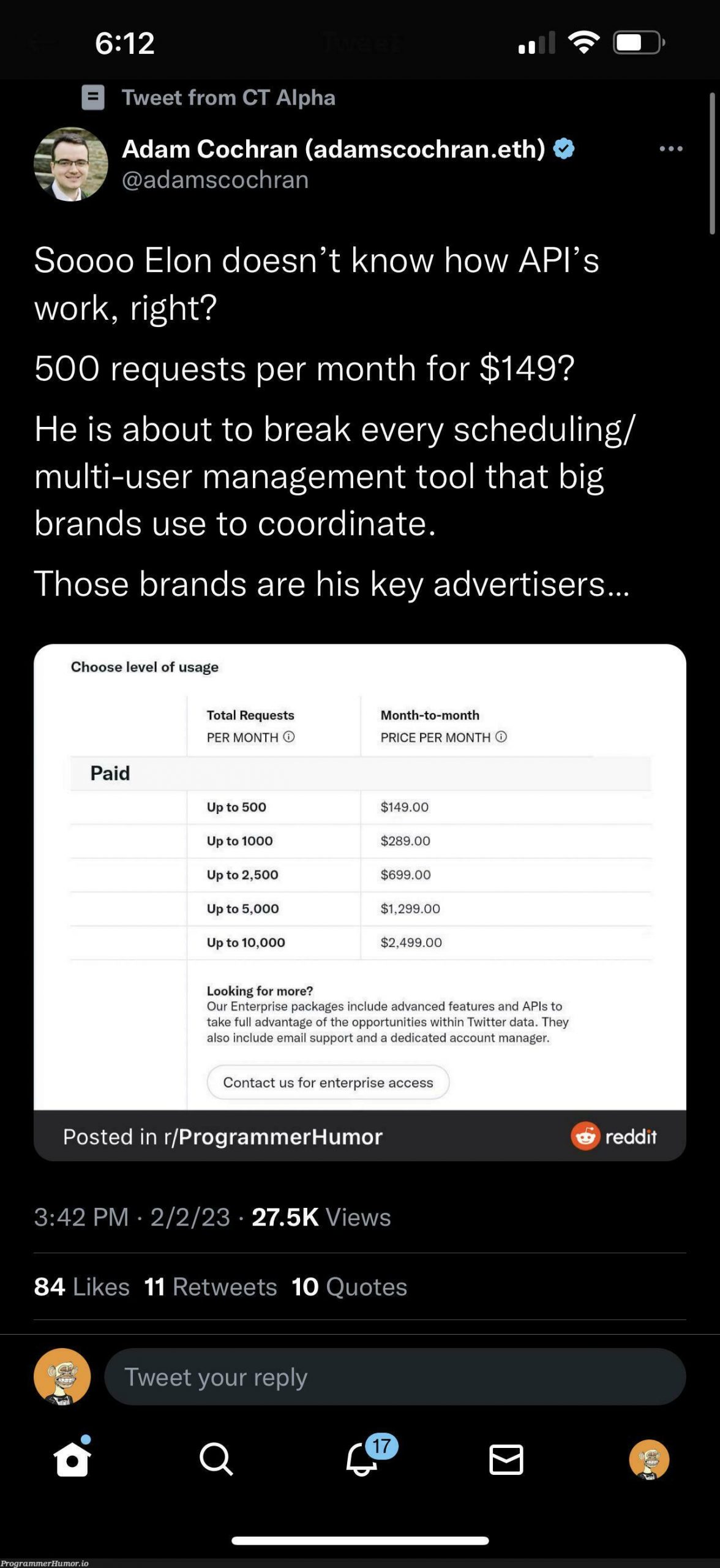**Caption:**

This image shows a smartphone screen displaying a tweet from @AdamsCochran.eth, criticizing Elon Musk's understanding of APIs. The tweet points out the high costs for API requests, stating that 500 requests per month cost $149, likely to disrupt crucial tools used by big brands, which are key advertisers. Additionally, the screen exhibits details of the API pricing structure in a white overlay box labeled "Choose Level of Usage." The pricing tiers are as follows: 

- Up to 500 requests per month: $149
- Up to 1,000 requests per month: $289
- Up to 2,500 requests per month: $699
- Up to 5,000 requests per month: $1,299
- Up to 10,000 requests per month: $2,499

The smartphone's status bar shows a moderate battery level, cellular signal with 2 bars, and Wi-Fi connectivity.